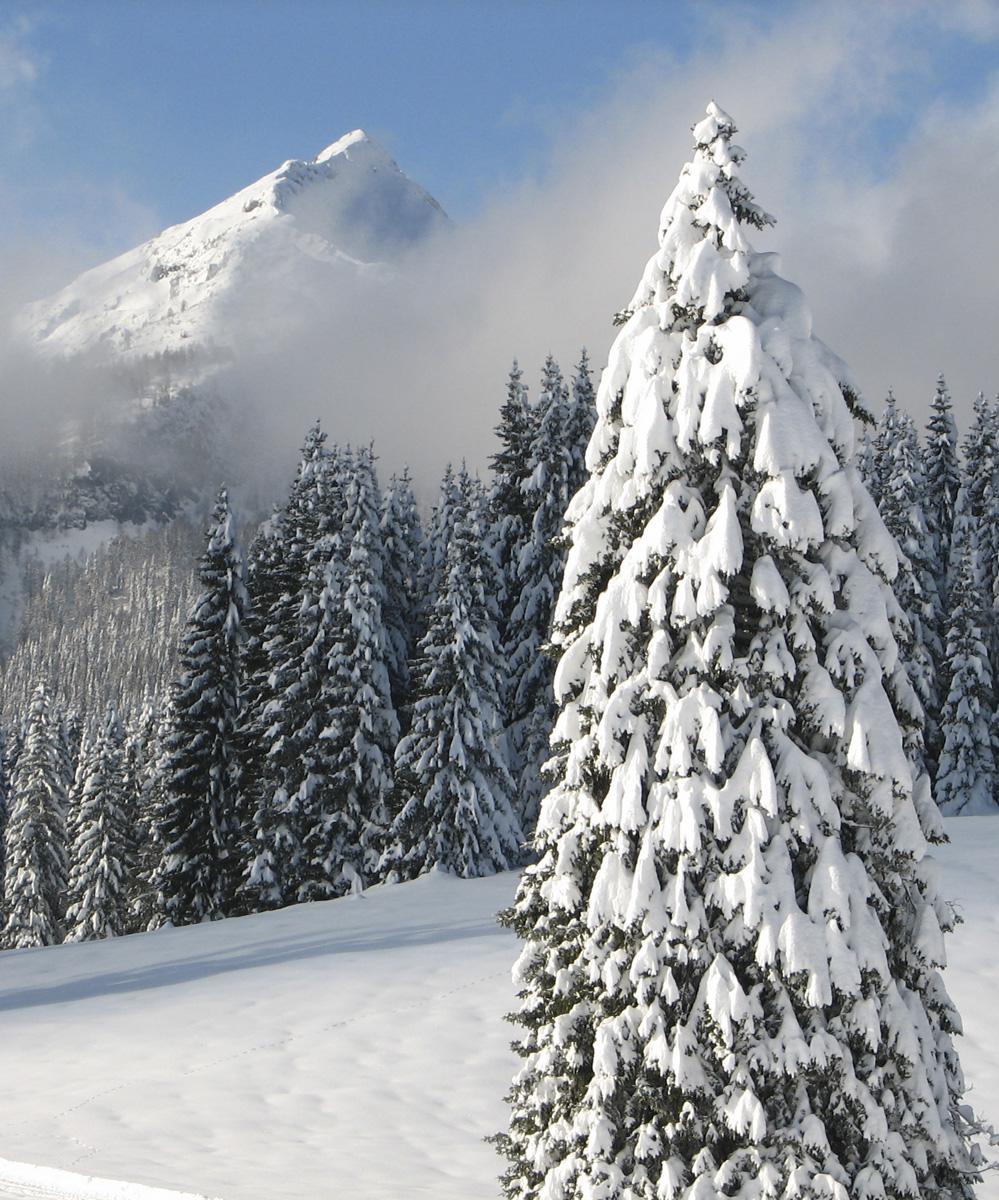This photograph captures a serene snow-covered landscape dominated by a tall evergreen tree, resembling a spruce or fir, in the foreground. The tree, elegantly coated in thick blankets of snow, gives the appearance of a grand ice cream cone with its slender branches bearing the weight of several inches of snow, although patches of green peek through. Extending beyond this stately tree is a large, untouched snowy slope leading to a dense forest of similarly snow-covered evergreens in the mid-ground. Among this backdrop, a layer of fog or mist subtly blankets the scene, adding a mystical haze. Rising majestically in the upper left corner is a snow-capped mountain, its contrast enhanced by a darker depression on one side, suggesting shelter from the snow. The mountain's peak, along with the rest of the pristine landscape, lends a sense of untouched wilderness to the photograph.